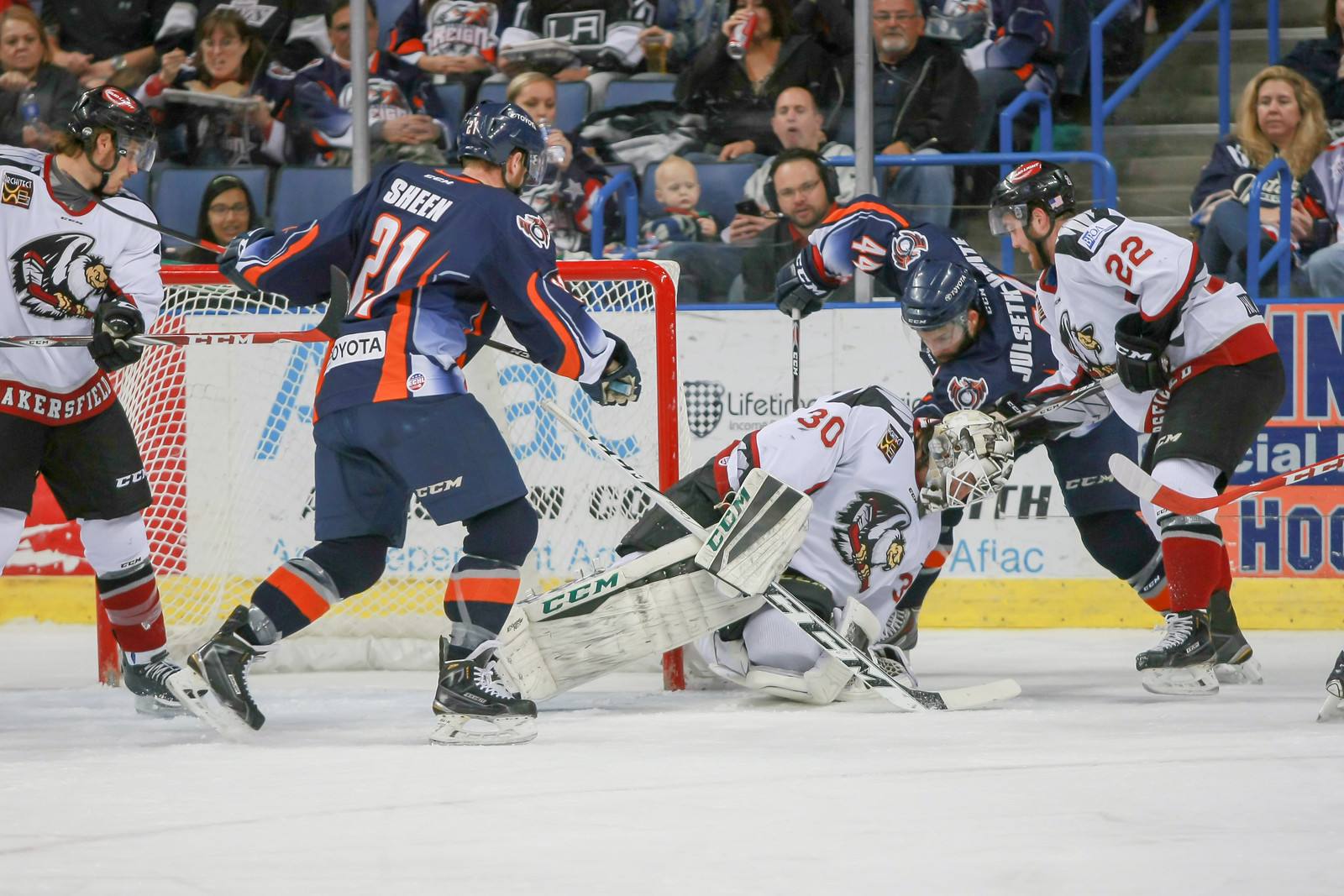This image captures a dynamic hockey match in action. The primary focus is on five players positioned near the goal. Two players from one team are dressed in blue long-sleeved jerseys, blue shorts, blue and white striped socks, black skates, and blue helmets. Notably, one player’s jersey, marked with "Sheen" and the number 21, stands out. 

Their opponents are clad in predominantly white jerseys with red accents and a distinct emblem resembling either an eagle or vulture. These players wear black shorts, white leggings, red socks, and black helmets, with their goalie sporting a white helmet and the number 30. The goal to the left is marked in red, suggesting an imminent attempt to score.

Beyond the rink, spectators of varying ages occupy blue seats behind the protective glass, intently watching the game unfold. The background is peppered with signs, contributing to the bustling atmosphere of the arena.